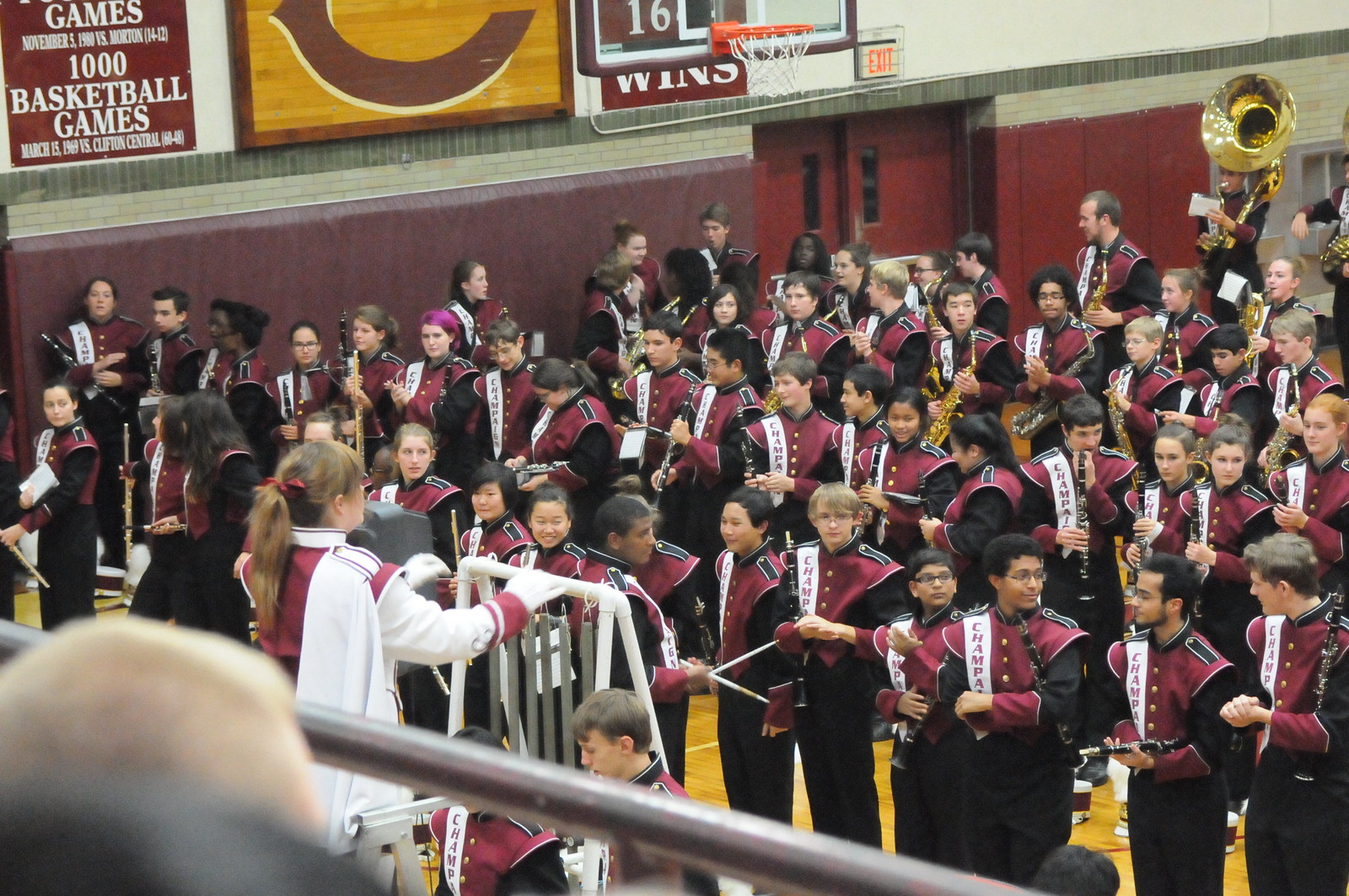This photograph captures a high school marching band in what appears to be a rehearsal or just before a show inside a school gymnasium, which doubles as an auditorium. The gym walls are adorned with various posters and banners about basketball games, indicating the multipurpose use of the space. The band members, a mix of male and female teenagers, are dressed in striking uniforms: purple torso with black shoulders, black sleeves, black pants, and purple wrists. Many members are holding their instruments, including trumpets, saxophones, flutes, and drumsticks, seemingly at ease, awaiting further instructions. At the center of the scene stands the conductor, a blonde girl elevated on a white podium. Her uniform features a distinctive design with a white base, white gloves, and purple accents on the torso, contrasting with the band's uniforms. She gestures authoritatively with her arms raised, likely calling the band to attention. The overall atmosphere suggests a moment of anticipation and readiness within the familiar setting of their school's gym.